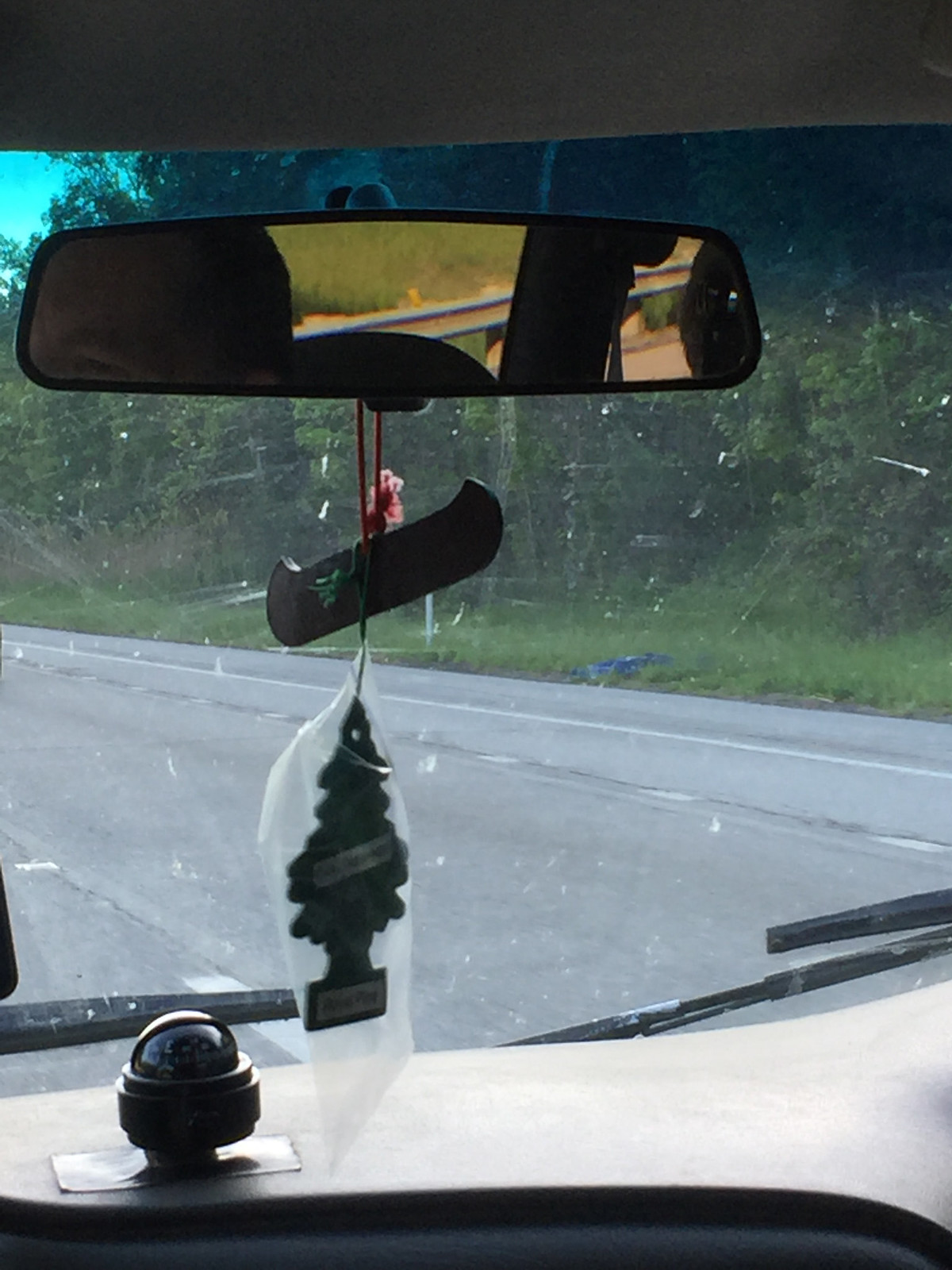The photograph captures the interior of a car from a passenger's perspective, taken through the dirty, chipped windshield. The view encompasses part of the dashboard, which prominently features a spherical stick-on compass. Hanging from the rear-view mirror are two decorations: a Christmas tree-shaped air freshener wrapped in plastic, and a small, black canoe-shaped ornament. The top of the driver's head is barely visible, shrouded in darkness. Outside, the car appears to be moving along a road lined with a green tree bank, driving on the left-hand side, suggesting a country where this is customary.